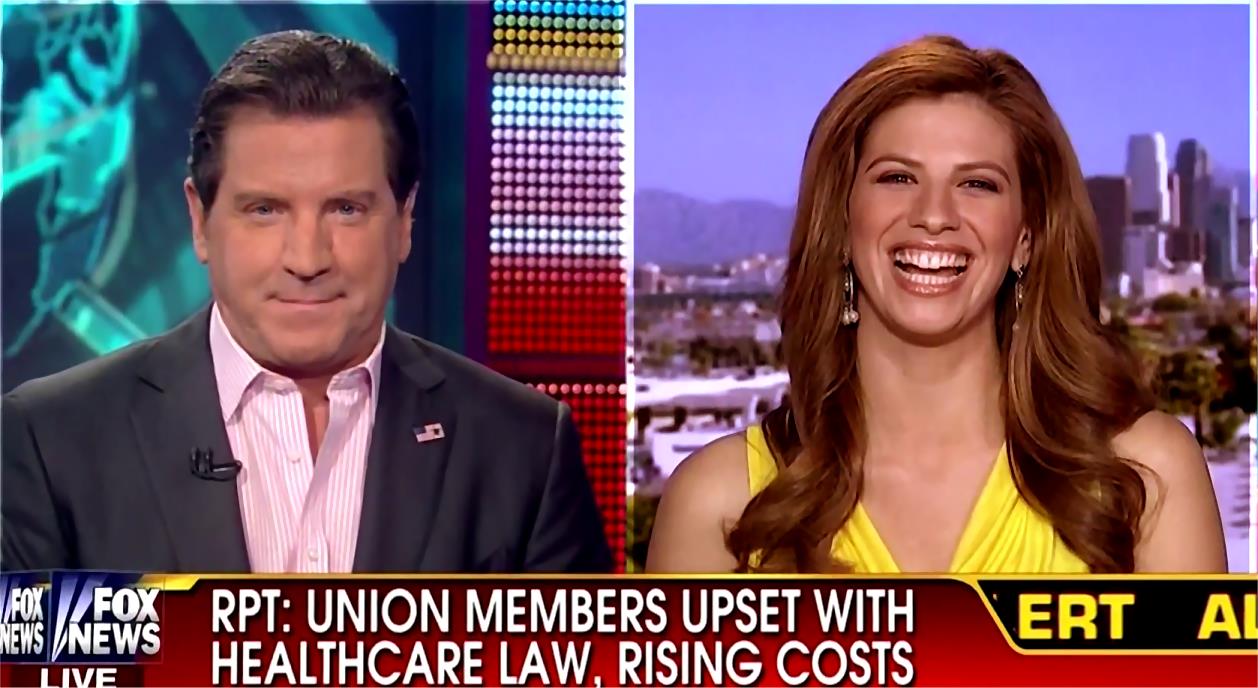The image is a live broadcast on Fox News, featuring a headline that reads "Report: Union Members Upset with Health Care Law, Rising Costs." An alert banner is displayed across the bottom. On the left, a male broadcaster is shown in a studio. He is wearing a gray suit with an American flag pin on his lapel and a light pink, striped shirt, which has the first button open. He has short dark hair and holds a microphone. Next to him, there is a woman with long red, shoulder-length hair who is smiling and wearing earrings and a yellow dress. She appears to be outside, standing in front of a backdrop depicting a cityscape. The two are engaged in conversation, with the woman likely being interviewed about the ongoing situation.